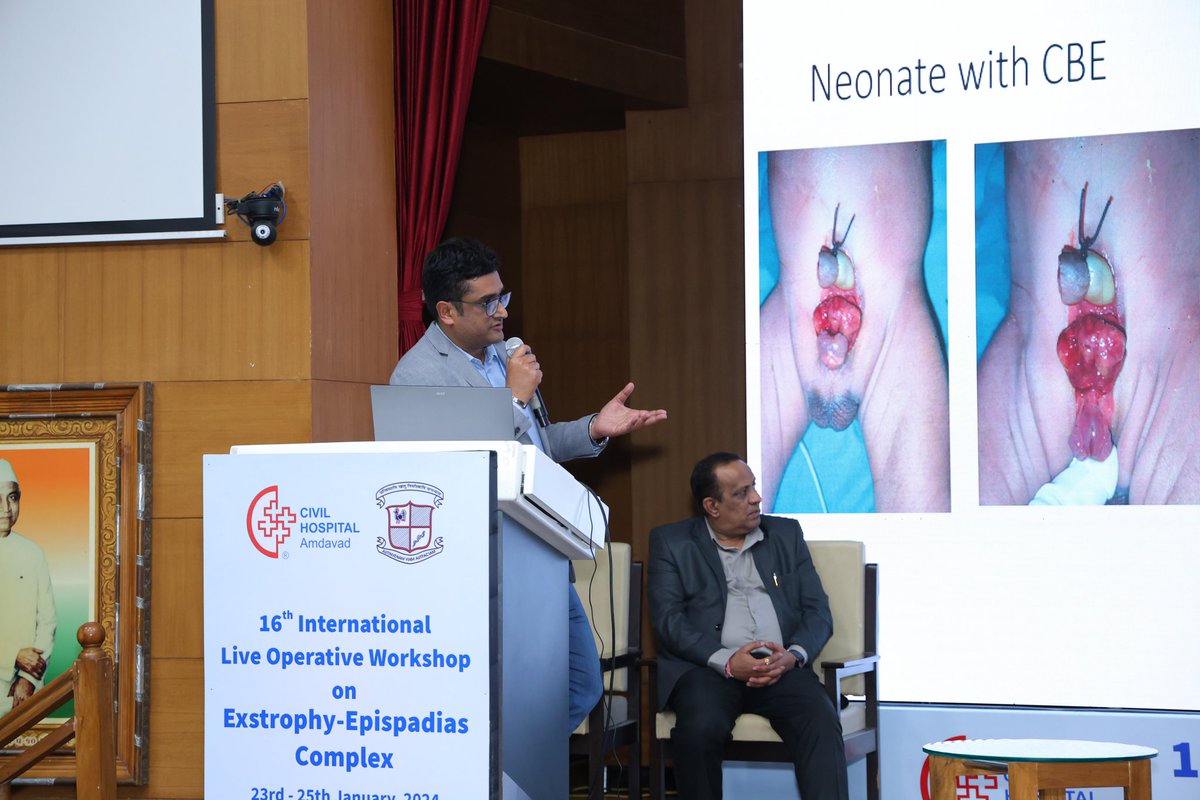This photograph captures a moment at the 16th International Live Operative Workshop on Extrophy Epispadias Complex, held from January 23rd to 25th, 2024. A man in a suit and glasses, likely the presenter, stands at a podium adorned with a microphone and a laptop. The podium features the logo and text from Civil Hospital Ahmedabad. He is elucidating images projected on the right side, showing graphic surgical details of male and female genital anatomy, including what appears to be a neonate undergoing surgery, labeled "Neonate with CBE." Below the projector screen sits another man, possibly an assistant or an observer, attentively watching the presentation. This detailed setup vividly captures the intensity and focus of a specialized medical workshop.